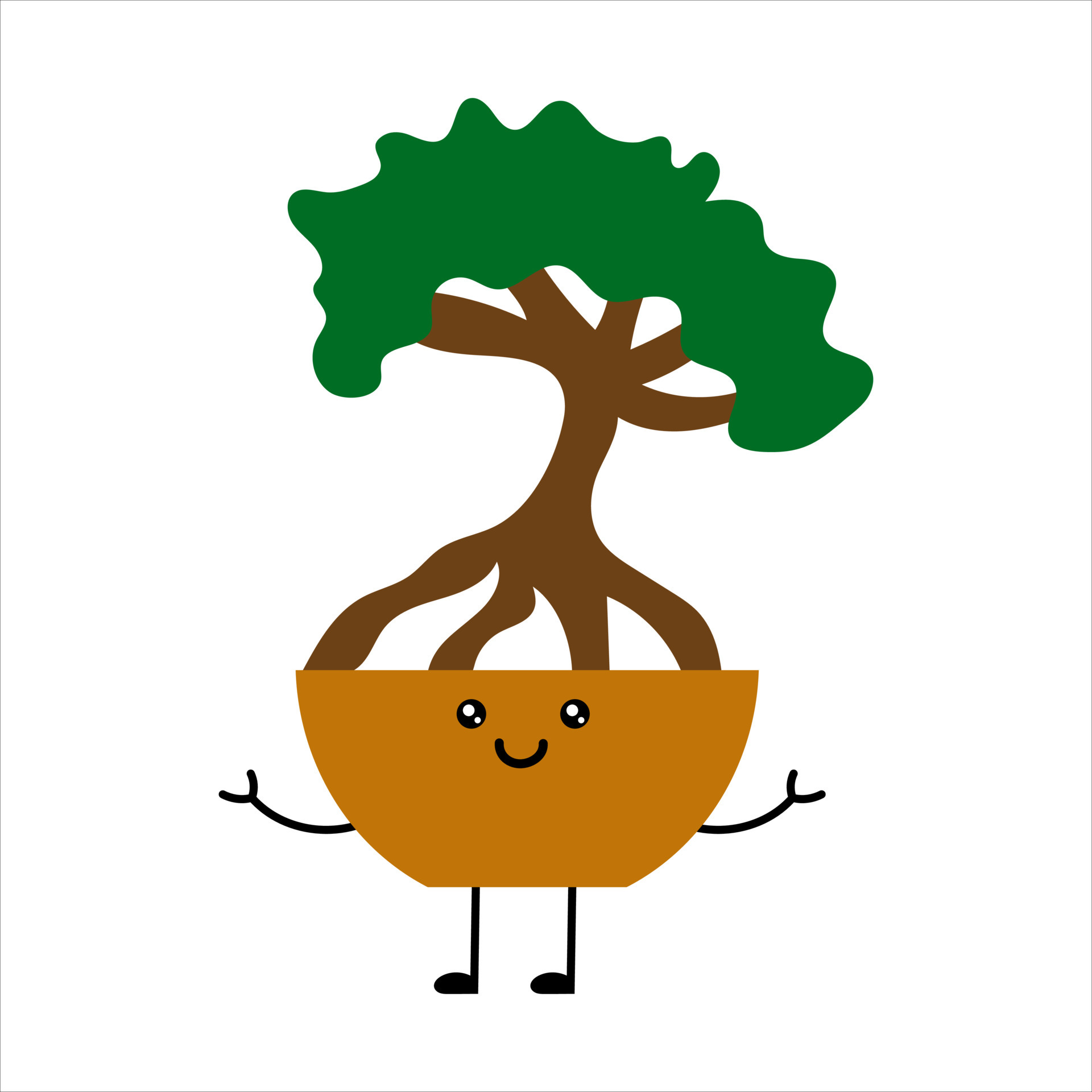The image is a simplistic digital art illustration of a charming character designed to look like a cup or a brownish-copperish bowl planter. The planter has a cute, emoji-like face with shiny eyes that include little white specks and a smiling mouth. From the top of the planter, tree roots emerge, transitioning into a larger tree with a brown trunk and branches supporting a mass of green leaves. The character also has stick figure limbs—black arms with tiny fingers and black legs with small feet—spreading out in a playful manner. The entire scene is set against a plain white background, adding to its childlike and elementary school drawing charm.